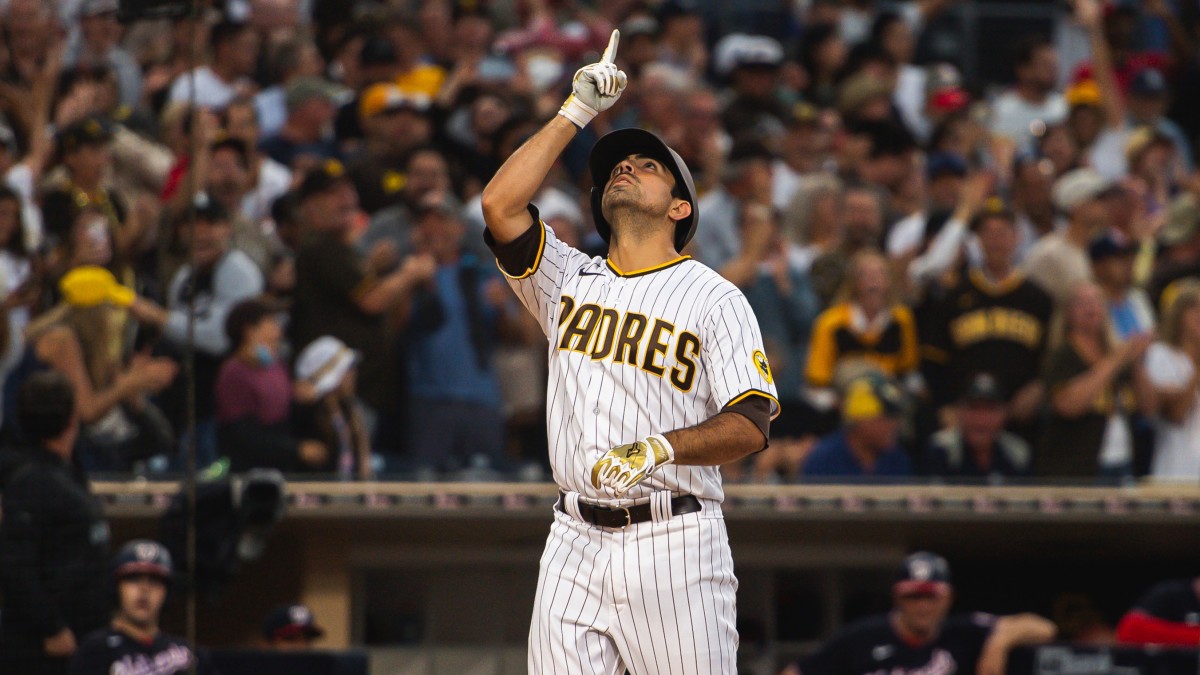The photograph features a baseball player prominently positioned in the center of the frame, donning the iconic uniform of the San Diego Padres. The uniform is distinctively white, adorned with vertical stripes that are either black or brown, providing a classic contrast. Underneath the jersey, he sports a shirt that complements the stripe color, likely black or brown. A vivid yellow circle logo is emblazoned on one sleeve, matching the yellow lining that trims the shirt. The word "Padres" is proudly displayed across his chest, outlined in the same striking yellow. 

The player's ensemble includes a black belt cinched at the waist, adding a functional and stylish touch. His head is protected by a baseball helmet, ensuring safety as he engages in the game. The player's gloves are an intricate blend of white, yellow, and gray, showcasing both style and utility. Capturing a moment of intensity and focus, he gazes skyward with a raised arm, pointing upwards as if signaling to the heavens. This pose captures the spirit and determination of the athlete, frozen in a moment of aspiration and reverence.